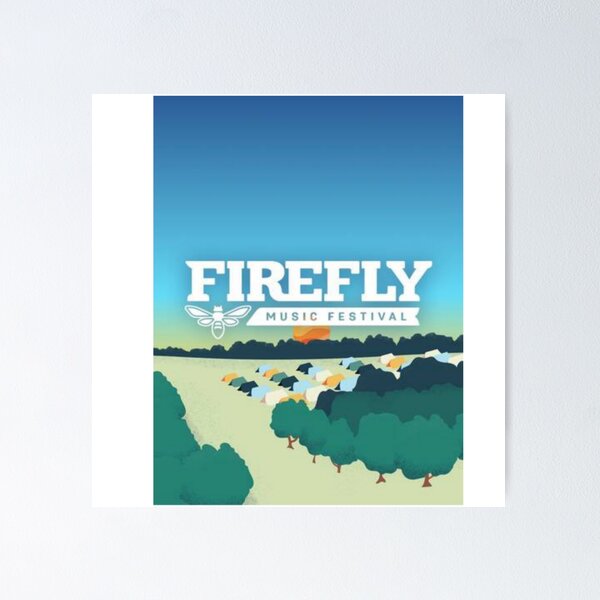The image portrays a meticulously designed poster for the Firefly Music Festival. Set against a light gray or whitewashed wall, the poster emulates a sheet of paper with a subtle drop shadow, enhancing its three-dimensional feel. The illustration within the poster has thick white borders on the sides, lending a letterbox effect. Dominating the scene is a serene, grassy clearing surrounded by rows of trees, extending from the lower left and right sides to the horizon where more trees and a setting sun are visible.

In the middle of this verdant clearing, colorful tents—orange, light green, dark green, light blue, and beige—are neatly lined up. Above this vibrant landscape, the sky transitions from blue to shades of green and yellow as it nears the treeline, creating a picturesque sunset. Superimposed against this scenic backdrop is the logo for Firefly Music Festival. "FIREFLY" in all caps stands prominently at the top, accompanied by "Music Festival" in a ribbon banner below, both in white text. A minimalist line drawing of a firefly with its wings outspread complements the logo, perfectly encapsulating the whimsical and natural essence of the festival.